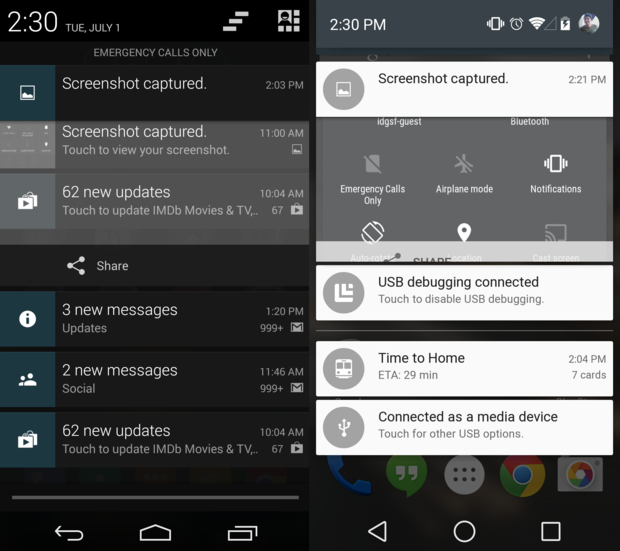This image consists of two horizontally aligned smartphone screenshots. Each one provides a glimpse into various details and notifications on the device.

**Left Screenshot:**
- **Top Section:** The time is displayed as 2:30 PM on Tuesday, July 1st, with a square profile icon on the right-hand corner.
- **Center:** The phrase "Emergency Calls Only" is prominently noted below the time.
- **Notifications:**
  - **Screenshot Captured** at 2:03 PM.
  - **Screenshot Captured - Touch to View Your Screenshot** at 11:00 AM.
  - **62 New Updates - Touch to Update IMDb, Movies and TV** at 10:04 AM.
  - **Three New Messages** under the category Updates at 1:20 PM.
  - **Two New Messages** under the category Social at 11:46 AM.
  - **62 New Updates - Touch to Update IMDb, Movies, and TV** repeated at 10:04 AM.
  - A Share icon is visible among the notifications.

**Right Screenshot:**
- **Top Section:** Also shows the time as 2:30 PM. Additional icons include a vibrating phone, alarm clock, WiFi connection, battery indicator, and a round profile picture.
- **Notifications (Horizontally Across the Page):**
  - **Screenshot Captured** at 2:21 PM.
  - **USB Debugging Connected - Touch to Disable USB Debugging** at 2:21 PM.
  - **Time to Home ETA 29 minutes** at 2:04 PM.
  - **Connected as a Media Device - Touch for Other USB Options** at 2:04 PM.

The detailed array of notifications and timestamps in both screenshots provide an insightful look into the device's activity and various prompts present at 2:30 PM on this particular Tuesday.